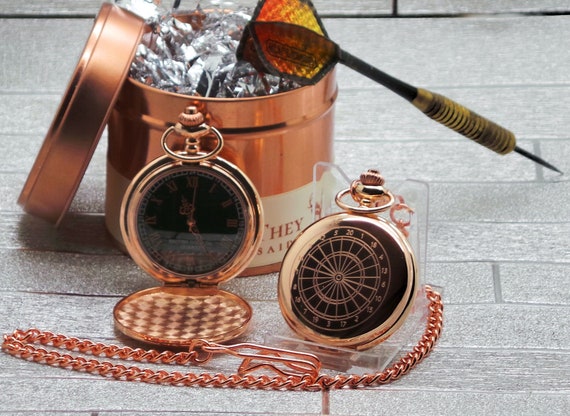This detailed photograph captures an assortment of luxury items, predominantly in opulent shades of copper and rose gold. In the foreground, two exquisite pocket watches with intricate black faces and delicate bronze-colored etchings sit prominently. One pocket watch features Roman numerals, while the other mimics the appearance of a dartboard with numbers 1 through 20 around its periphery. Both watches are open, revealing their intricately designed inner covers.

Just behind these elegant timepieces is a copper-colored canister, resembling an ice bucket, with its lid removed and placed to the side. The interior of the canister is lined with silver foil, adding a reflective quality to the scene. Resting against this canister is a black dart with striking orange and yellow fins, adding a touch of sporty flair to the luxurious setup.

All the items are arranged on a surface that appears to be silver-gray in color, possibly a dove gray vinyl or tile floor, contributing to the sophisticated and polished aesthetic of the image.